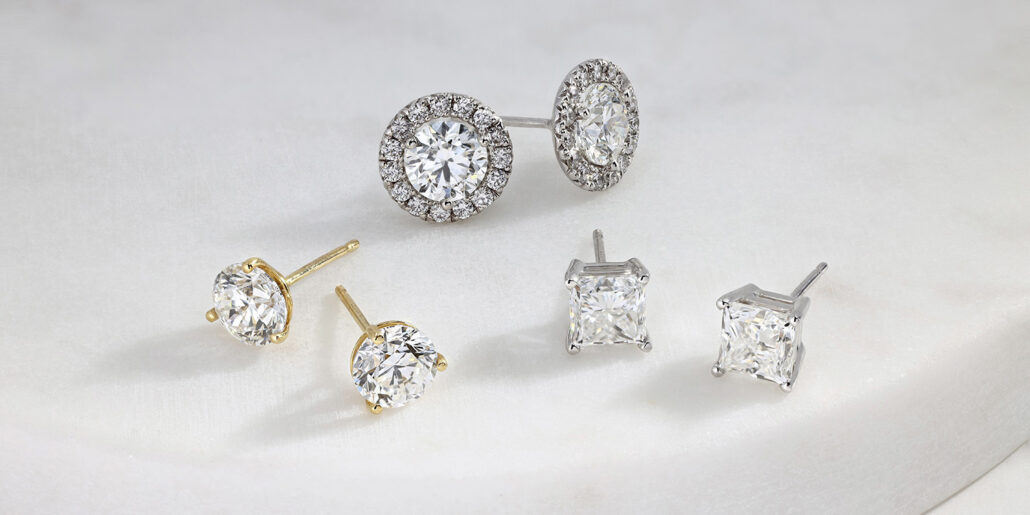This rectangular photograph showcases three pairs of stud earrings beautifully arranged on a pristine white background, reminiscent of a clean white tabletop. Each pair of earrings features sparkling stones, likely diamonds or cubic zirconia, each set in its distinct metal setting. 

At the top, the largest studs are halo-style, crafted in silver or white gold. These earrings boast a central round diamond encircled by a halo of smaller diamonds, creating a sun-like appearance. 

In the lower right corner, there are square-shaped stud earrings, known as princess cut. They are set in a traditional four-prong setting, also in silver or white gold.

Finally, in the lower left, there's another pair of round stud earrings. These are distinguished by their gold prongs, posts, and stems, creating a striking contrast between the yellow gold and the clear, round diamonds. Although missing their backing in the image, all pairs are designed for pierced ears. The detailed craftsmanship of each earring pair highlights the timeless elegance and versatility of stud earrings in varying shapes and metals.